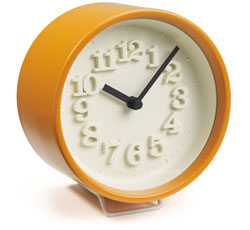The image features a small, round clock with a distinctive design. The clock is supported by a wireframe base painted in an off-white color. The housing around the clock is a vibrant orange, adding a pop of color to its appearance. The clock face is stark white, adorned with raised white numerals which are clearly visible due to the shadows cast by the numbers. The minute and hour hands are black, providing a sharp contrast that makes them easy to read. The clock is showing the time as approximately 10:08. Beneath the clock, the surface reflects the orange hue from its housing, adding a subtle glow. The clock face is minimalistic, featuring no other markings or writing aside from the raised numerals. Between each hour numeral, there are small tick marks that further aid in time reading.